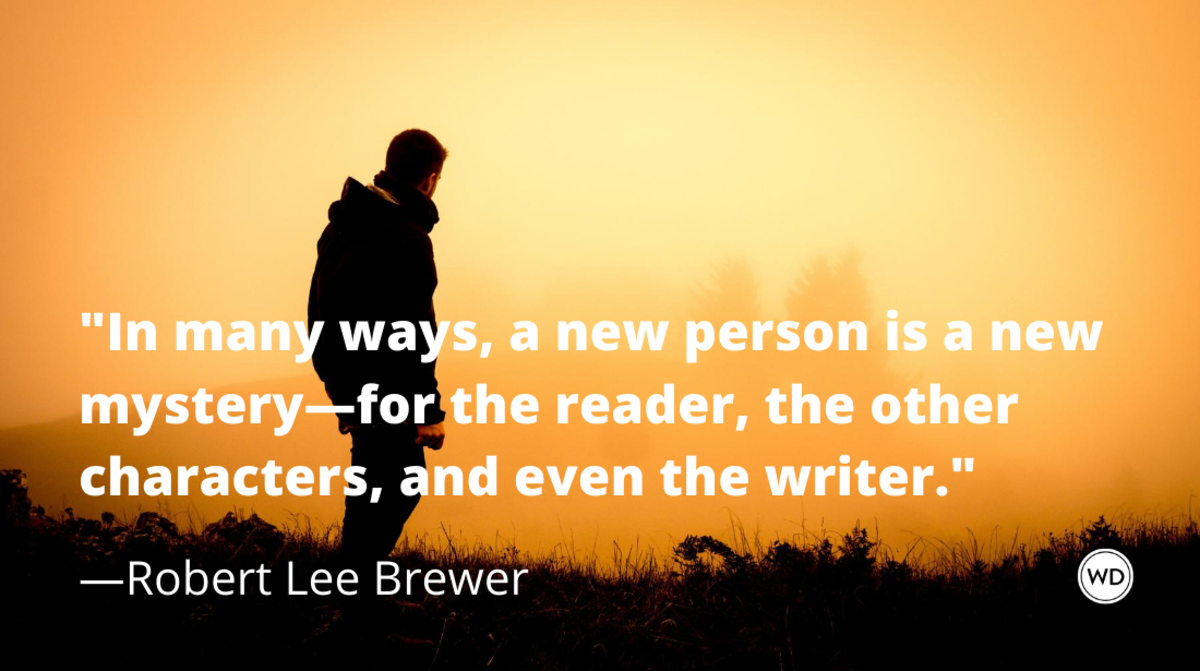The image depicts a striking scene set against an orange gradient sky, resembling a sunset, where a silhouetted man stands in a field of dirt with small plants and grasses. The man is turned slightly to the side, revealing some details like the lighter coloring on his face, ear, and right hand. He is dressed in a dark coat with a hood and long pants. Overlaid on this silhouette is a quote in white text: "in many ways, a new person is a mystery for the reader, the other characters, and even the writer." At the bottom center of the image, the quote is attributed to Robert Lee Brewer, and in the bottom right corner, there is a white circle with the letters "W.D." in dark text. The overall composition blends the warm tones of the sky with the stark contrast of the silhouetted figure to create a contemplative and evocative scene.